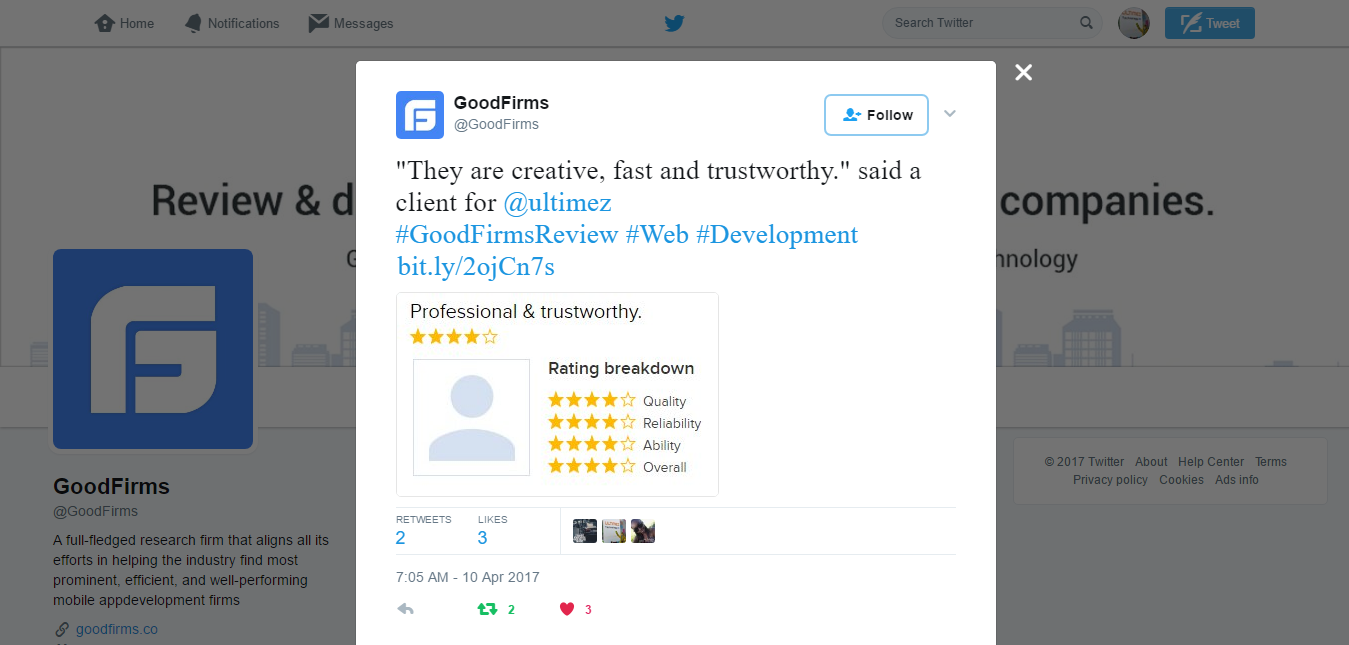The image features a gray background with several interface elements at the top, including icons for home, Netflix, and messages, alongside a small blue bird icon. Beneath these icons, there is a search bar followed by a circular icon containing white elements. Additionally, a blue button for email is present.

In the center of the image, there is a prominent white box featuring a blue rectangle with a large white 'G', labeled "GoodFirms." Below this, there is a blue follow button accompanied by a client testimonial stating, "They are creative, fast, and trustworthy - a client for Ultimate," followed by hashtags #GoodFirmsReview, #Web, #Development, and a shortened URL, bit.ly/toOJCIN7. 

A rating breakdown is displayed, showing four stars across categories like quality, ability, and overall reliability. Next to these, there are small icons: a box with numbers '2' and '3', three small thumbnail pictures, a timestamp of 7:05 AM, a left arrow, and some green arrows. There is also a red heart icon with the number '3' beside it. The gray background is partially visible around the central elements.